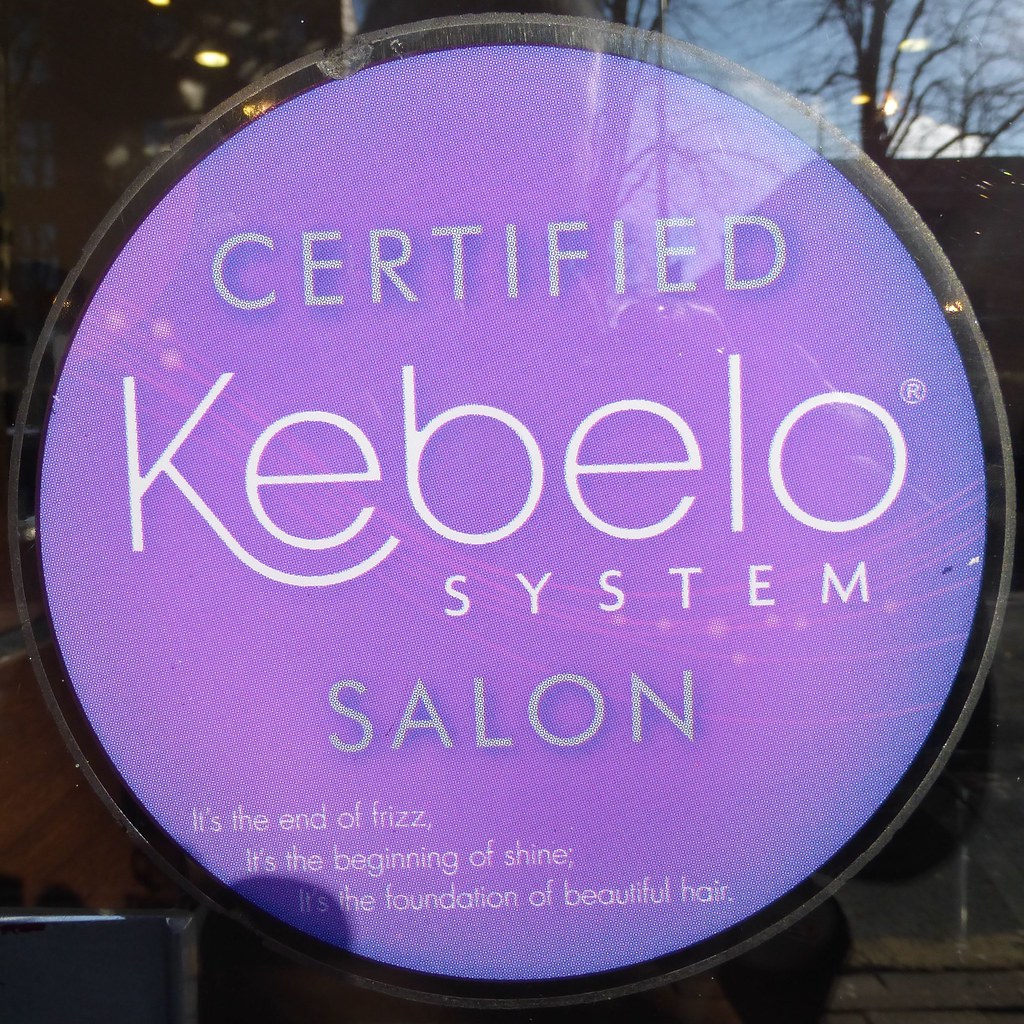The photo captures a storefront window featuring a prominent, illuminated circular sign with a purple hue and a black frame. The sign reads, in descending order, "CERTIFIED" in gray capital letters, "Cabello System" in white, "SALON" in gray capitals, and a tagline in light gray stating, "It's the end of frizz, it's the beginning of shine, it's the foundation of beautiful hair." The sign has a small circular trademark symbol next to "Cabello," and the purple color glows softly. Reflections on the window reveal the photographer, along with trees, houses, and sky in the background, adding depth to the image. The shadow of the person taking the picture is visible in the lower left-hand corner, further enhancing the layered composition.